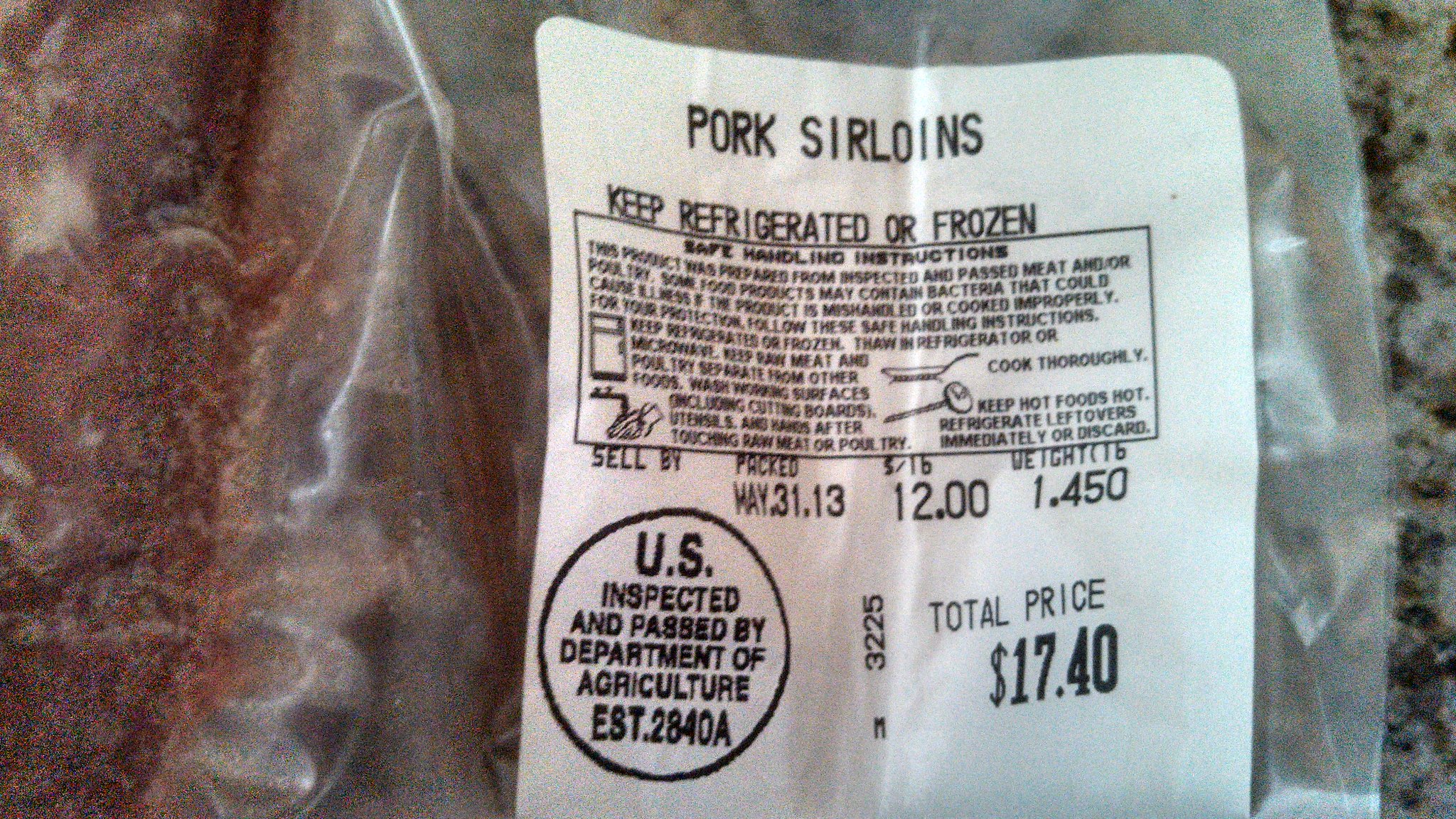Close-up of a pack of frozen pork sirloins placed on a kitchen counter. The countertop, made of granite, is partially visible on the right. The main focus of the image is a transparent plastic bag containing the frozen meat, which has a dark reddish hue. A white label on the left-hand side of the bag provides detailed product information. The label reads: "Pork Sirloins. Keep refrigerated or frozen." It also includes safe handling instructions, a sell-by date (which is not filled in), and additional details such as weight and price. The packed weight is marked as .31 and .13 pounds, with a unit price of $12 per pound and a total weight of 1.450 pounds. At the bottom left of the label, a circular stamp indicates that the product has been inspected and passed by the U.S. Department of Agriculture, establishment number 2840A, along with the identifier M3225. The total price of the pack is $17.40.